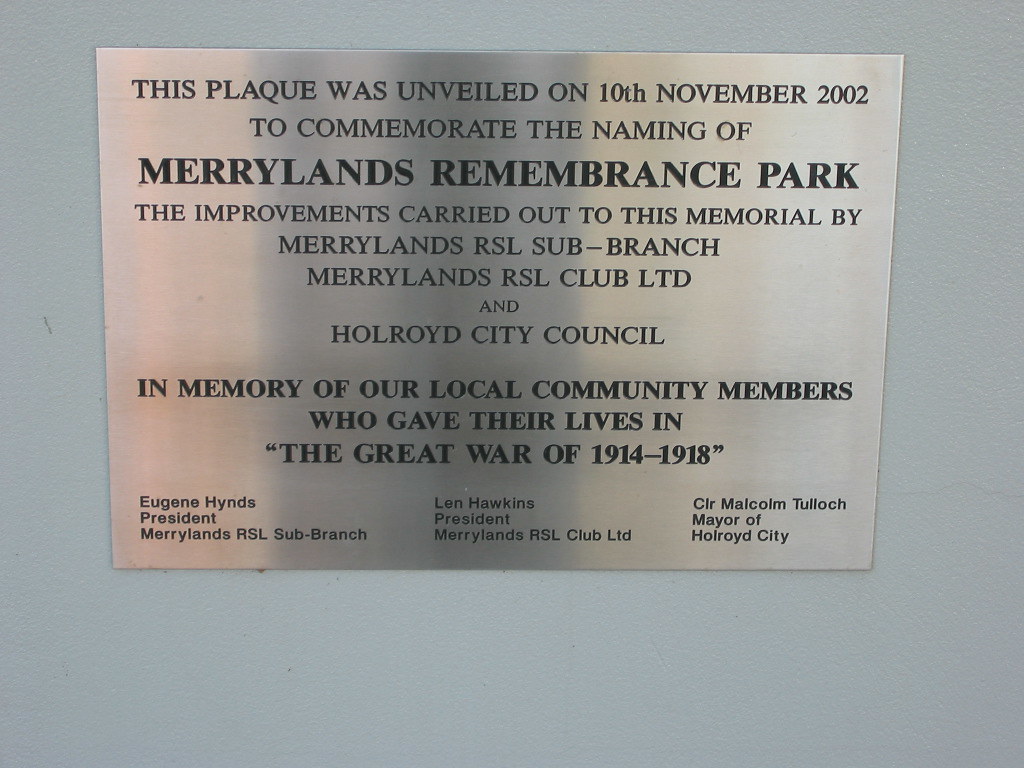This photograph captures a detailed image of a silver metal plaque mounted on a predominantly white wall. The plaque prominently displays black, capitalized, and centered text. It reads: "THIS PLAQUE WAS UNVEILED ON 10TH NOVEMBER 2002 TO COMMEMORATE THE NAMING OF MARYLAND’S REMEMBRANCE PARK." Below this, in a smaller and less bold font, it details: "THE IMPROVEMENTS CARRIED OUT TO THIS MEMORIAL BY MARYLAND’S RSL SUB-BRANCH, MARYLAND’S RSL CLUB LTD, AND HOLROYD CITY COUNCIL." The inscription then highlights in bold: "IN MEMORY OF OUR LOCAL COMMUNITY MEMBERS WHO GAVE THEIR LIVES IN THE GREAT WAR OF 1914 TO 1918." The bottom section lists key individuals associated with the memorial, in smaller text each on its own line: "EUGENE HINES, PRESIDENT, MARYLAND'S RSL SUB-BRANCH; LEN HAWKINS, PRESIDENT, MARYLAND'S RSL CLUB LTD; CLR MALCOLM TULLOCH, MAYOR OF HOLROYD CITY." The plaque stands as a solemn tribute to the community's history and the sacrifices made during the Great War.